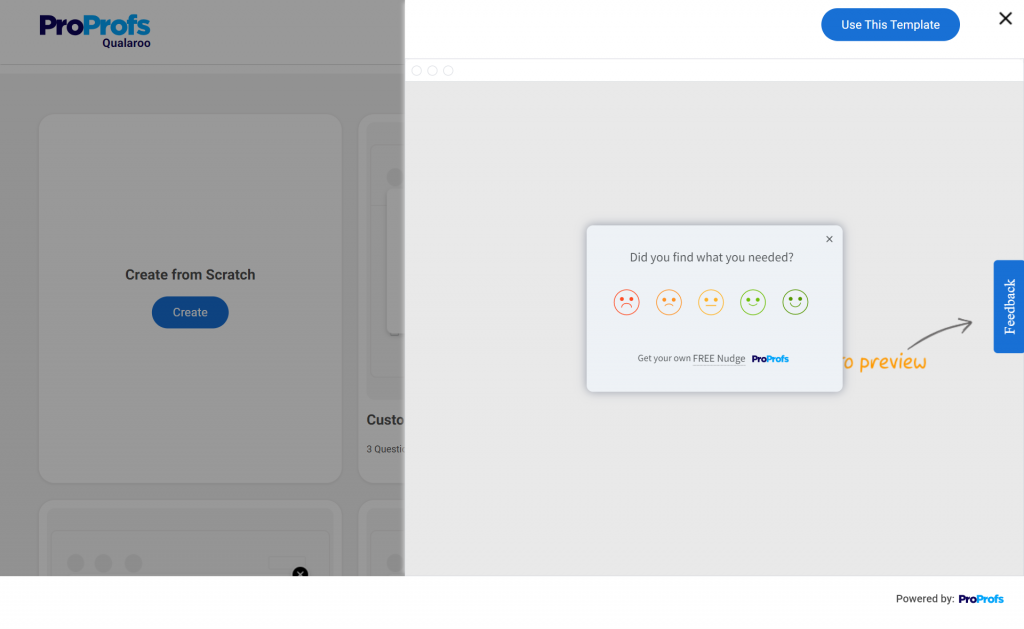The image showcases a webpage from a website called ProProfQualelru, which appears to specialize in offering templates. The layout is divided into two sections. 

On the left, the background is darker and slightly grayed out, displaying various template options. The heading here reads "Create from Scratch," accompanied by a prominent blue "Create" button. Behind this interface is a blank, white sheet indicating a new, empty template ready for customization.

The right side of the image features a lighter gray background and includes a blue "Use This Template" button with an 'X' symbol adjacent to it, suggesting the option to select or dismiss a particular template. This section also highlights a feedback feature, indicated by another blue button with an arrow.

A central dialog box is open, asking users "Find what you needed?" accompanied by five smiley-to-frowny faces in varying colors, ranging from very unhappy to very happy, for users to give quick feedback. Below this box, there's an advertisement stating "Get your own free nudge," likely promoting a service or additional feature available on the website.

At the very bottom of the image, in small text, the site indicates it is "Powered by ProProfs." ProProfQualelru appears to be a unique and specialized website dedicated to providing a variety of templates.